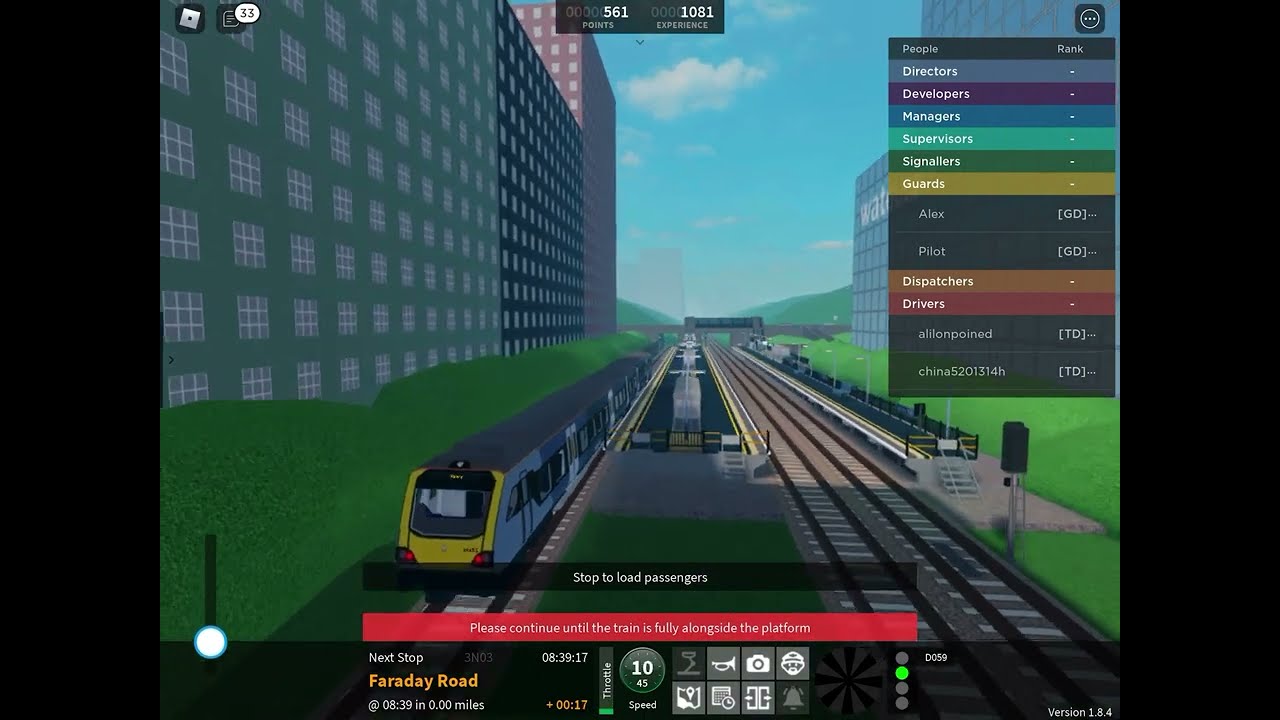The image is a detailed screenshot from a train simulator video game that captures a complex and immersive scene. The focus of the image is a bustling train station situated in a diverse environment that combines elements of urban and rural landscapes. On the left side, there are tall, 3D-rendered buildings in blue and green tones that stretch upwards, out of the frame, providing a modern, digital cityscape backdrop. Just beneath these structures are carefully detailed hedges and bushes, adding to the scenic realism.

In the center, two train tracks run into the distance, converging at an angle to create a sense of depth. On the left track, there's a sleek, silver-colored train with a black roof and yellow front, reminiscent of a metro or bullet train, complete with numerous windows. The right track lies empty, emphasizing the stillness of the platform, which is awaiting passengers. Surrounding the tracks are expansive green grassy areas that contribute to the laid-back, countryside vibe.

To the right, additional buildings rise towards the sky, offering a striking contrast with the greenery around them. The user interface (UI) overlays the scene, providing a wealth of information and interactive elements. A prominent menu on the right displays various roles such as Directors, Developers, Managers, Supervisors, Signalers, and Guards, along with names assigned to these roles—indicating a multiplayer aspect where users can assume different positions within the simulation.

At the bottom center, the UI indicates the train’s real-time speed, currently at 10 miles per hour, and includes control icons for the camera, horn, and map. Text instructions direct players to "stop to load passengers," and further specify, "please continue until the train is fully alongside the platform." Additional navigation elements display the next stop details, including time and location—Faraday Road, in 8 hours, 39 minutes, and 17 seconds.

Overall, this train simulator game offers a highly detailed and realistic experience where players manage passenger loading and train operation, all while navigating a richly designed virtual environment.